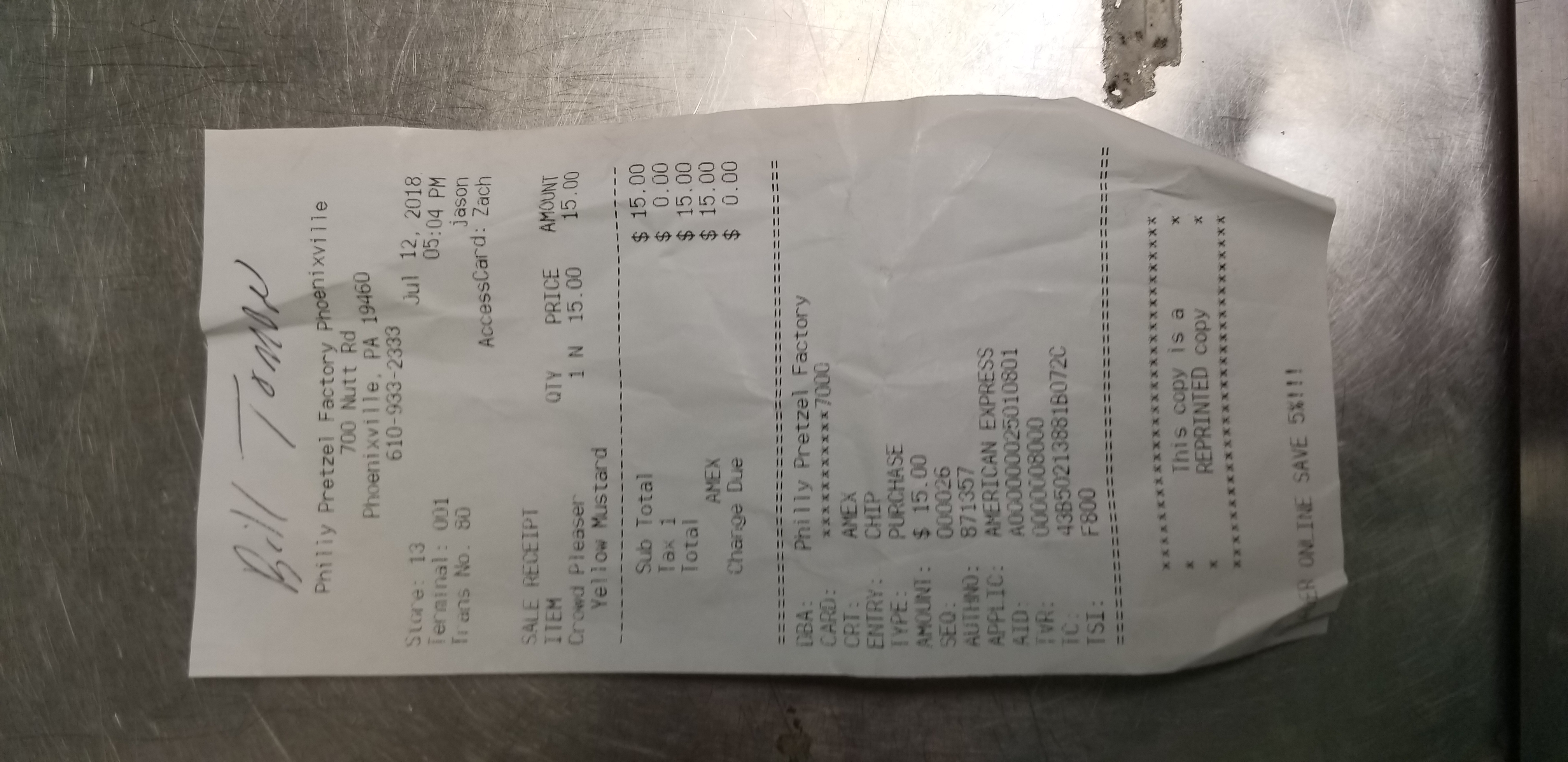The image depicts a black-and-white photograph of a receipt placed horizontally on a stainless steel counter. The receipt is white with black print, prominently featuring the name "Bill Tillman" and the establishment "Philly Pretzel Factory." Although partially obscured, the location information includes an address on "700 mil road" in a town ending with "ville" in Pennsylvania. The receipt's total purchase amount is $15, though the specific items bought are not discernible.